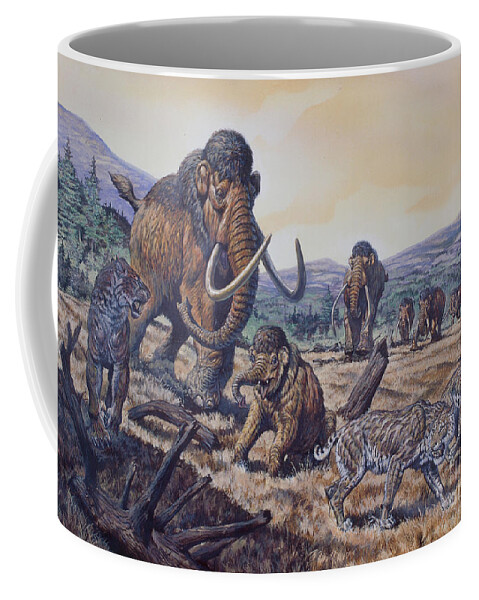This detailed photograph showcases a coffee mug set against a completely white background, emphasizing its painted artwork. The mug, with a white interior and white handle visible on the left side, features a detailed, almost antique-looking scene depicting a prehistoric era. The artwork wraps around the mug, portraying a barren, dry landscape with brown, dead grass and scattered sticks in the foreground. Adorning the scene are woolly mammoths; notably, an adult mammoth accompanied by a baby mammoth stands prominently in the center. The background reveals lush green trees and rugged brown mountains under a dusk-like, tan or rust-colored sky. Alongside the mammoths, various prehistoric animals are depicted, including large cats reminiscent of tigers or leopards. One of these cats is seen skulking away to the bottom right, while another snarls back at the baby mammoth on the left. The overall painted scene offers a nostalgic, dated quality, capturing a moment of quiet tension among the animals from a bygone era.